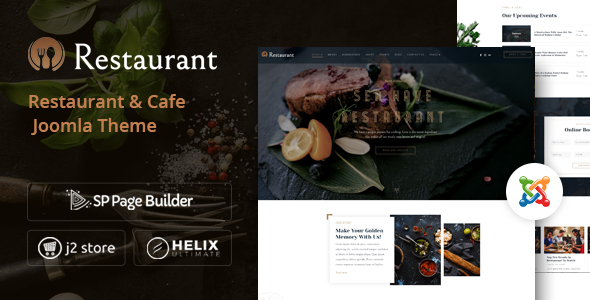This image is a screenshot from a restaurant website showcasing various web design elements and features. At the top, the word "Restaurant" is prominently displayed next to a logo featuring a fork and spoon on an orange background. Below this, in the same orange color, the text "Restaurant and Cafe Joomla Theme" is visible, indicating the type of web template being used. Adjacent to this, icons and labels such as "SP Page Builder" with a triangle and confetti design, "J2 Store" with a cart symbol, and "Helix" within a circle are present, illustrating the tools and extensions available.

On the right side of the image, there's a visually appealing photo of a gourmet meal—likely a steak or fillet—served on a black slate plate. This dish is garnished with lemon slices artfully arranged on a leaf, enhancing the presentation. The text "Sell Have Restaurant" overlays this food image, suggesting the name or feature of the restaurant being highlighted.

At the top right corner of the image, there are clickable areas, which are partially obscured by a pop-up showcasing the delicious meal. At the bottom of the screenshot, an article titled "Make Your Goldest Memory with Us" is partly visible, inviting further reading. Additional clickable options are also seen on the right, offering more navigation choices within the website.